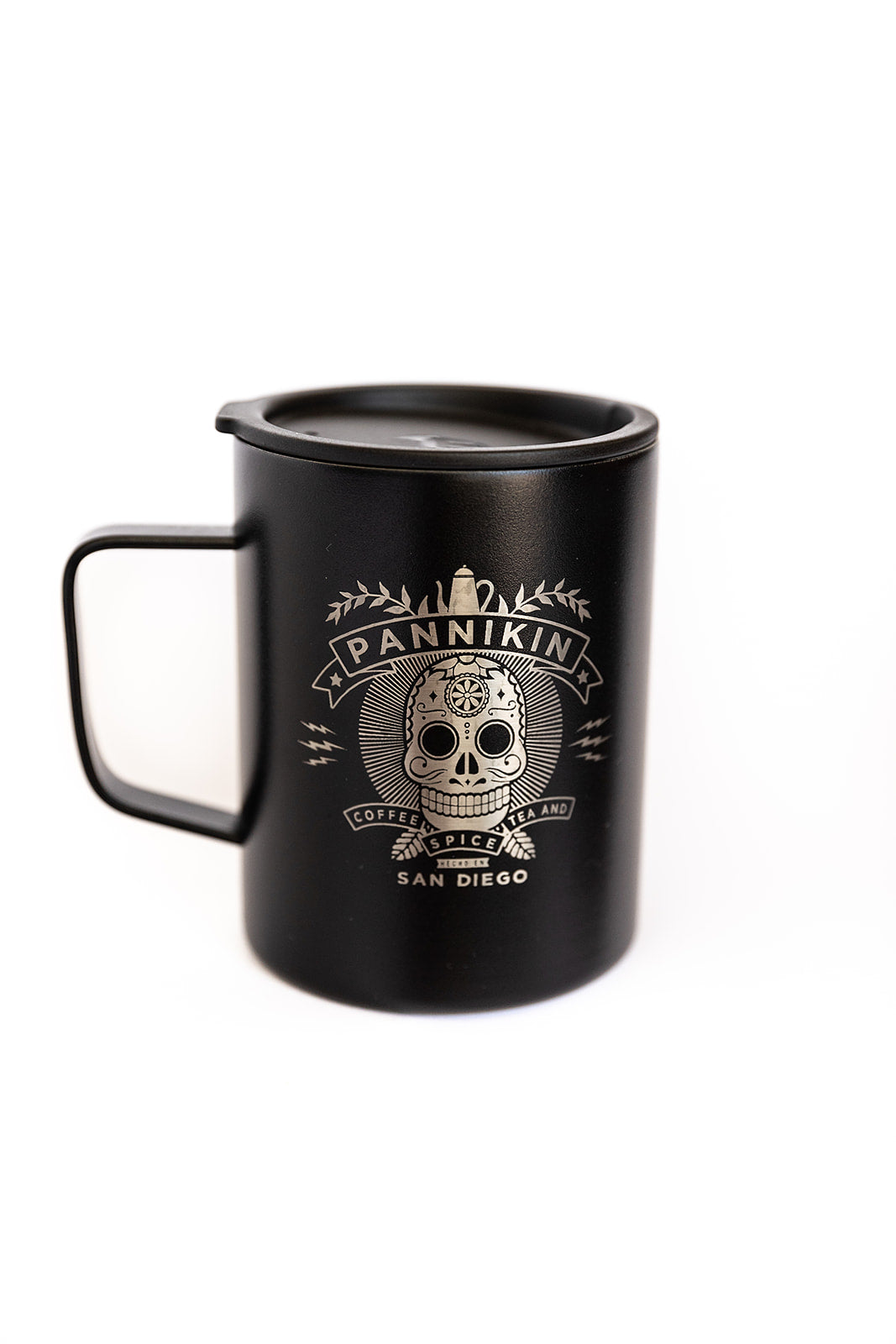This is an image of a medium-sized, glossy black travel mug adorned with an intricate design. The mug features a secure black lid to prevent spills, making it ideal for on-the-go use, whether in a car or on a walk. The front of the mug is decorated with a gold and silver-tone graphic of an ornate Mexican folk skull, complete with a flower design on its forehead. Surrounding the skull are detailed elements including lightning bolts on either side, and a halo-like arrangement of rays. At the top of the design, a small vintage teapot graphic sits above a banner that reads "Panikin." Beneath the skull, there are three banners that say "Coffee," "Spice," and "Tea." The smallest print, which is partially illegible, is located under the word "Spice." At the very bottom, in white text, it says "San Diego," referencing the location of the coffee company. The overall finish of the mug is slightly shimmery, adding an extra touch of elegance to its detailed design.